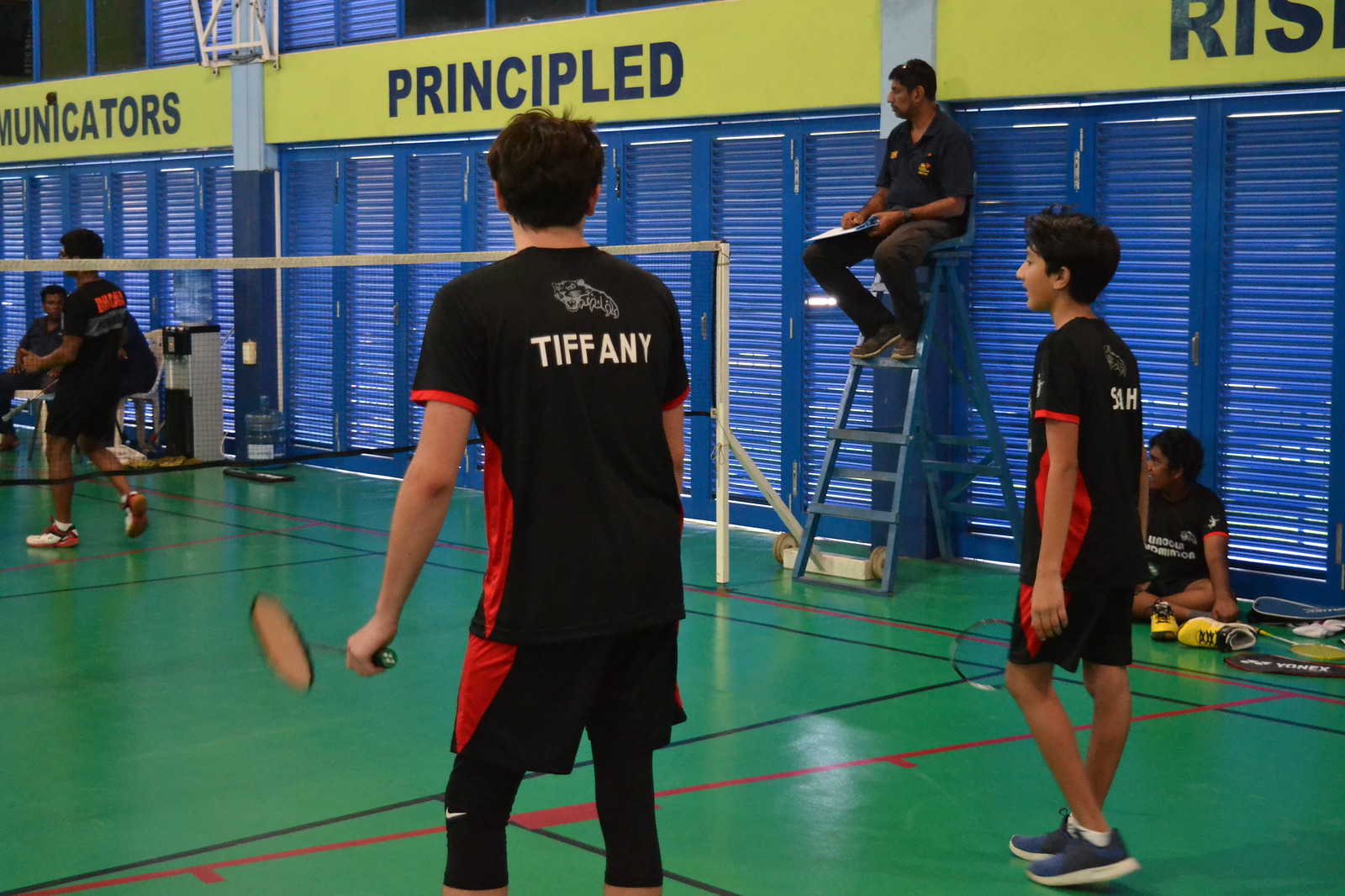In this vibrant photograph captured inside a gymnasium, a competitive game of badminton unfolds on a pristine green court lined with distinct black and red markings. The center of the field is dominated by a badminton net, with an umpire seated high atop a ladder, attentively monitoring the match. On one side of the net, two players clad in black t-shirts and shorts, accented with red designs, engage energetically; on the other side, a single player faces them. The visible player from the back reveals the name "Tiffany" on his jersey. 

Surrounding the court, spectators either stand or sit near the boundary, engrossed in the game's proceedings. One spectator is visibly removing his shoes while another appears to be in pursuit of hydration from a water dispenser. The gymnasium's walls exude a metallic blue hue, punctuated by a prominent yellow stripe emblazoned with blue text that references "Principled Communicators." This scene vividly captures the intense atmosphere and camaraderie common in competitive sports gatherings.